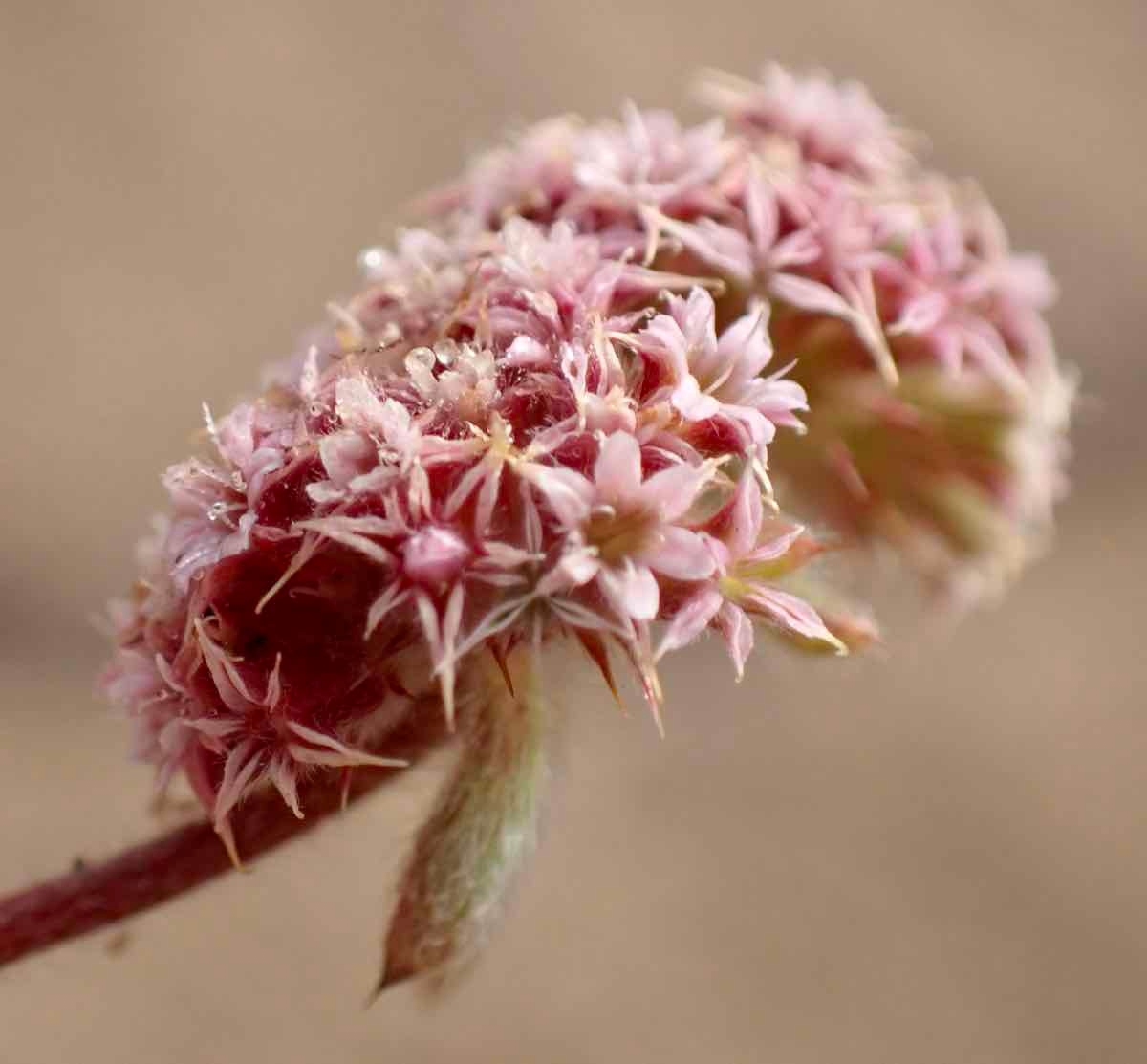This image captures a stunning close-up of a flower mid-bloom, prominently featuring a large cluster of small, star-shaped blossoms. The blooms, numbering around 40 to 50, exhibit a range of pink hues—deep pink at the center fading to almost white at the tips—indicating varying ages of the flowers. Some petals appear older and have lost much of their color. Dewdrops delicately adorn the petals, suggesting a recent rainfall. The flower's stamen is visible, with a fuzzy greenish tint, and there are also little green bits interspersed among the blooms. A slightly hairy leaf extends from the bottom of the cluster. The blurred background, in shades of brown and tan, highlights the flower in sharp focus, with the stem curving up from the left and appearing as a dark purple-pink color. This vivid, detailed image emphasizes the flower’s vibrant colors and intricate details against a softened backdrop.